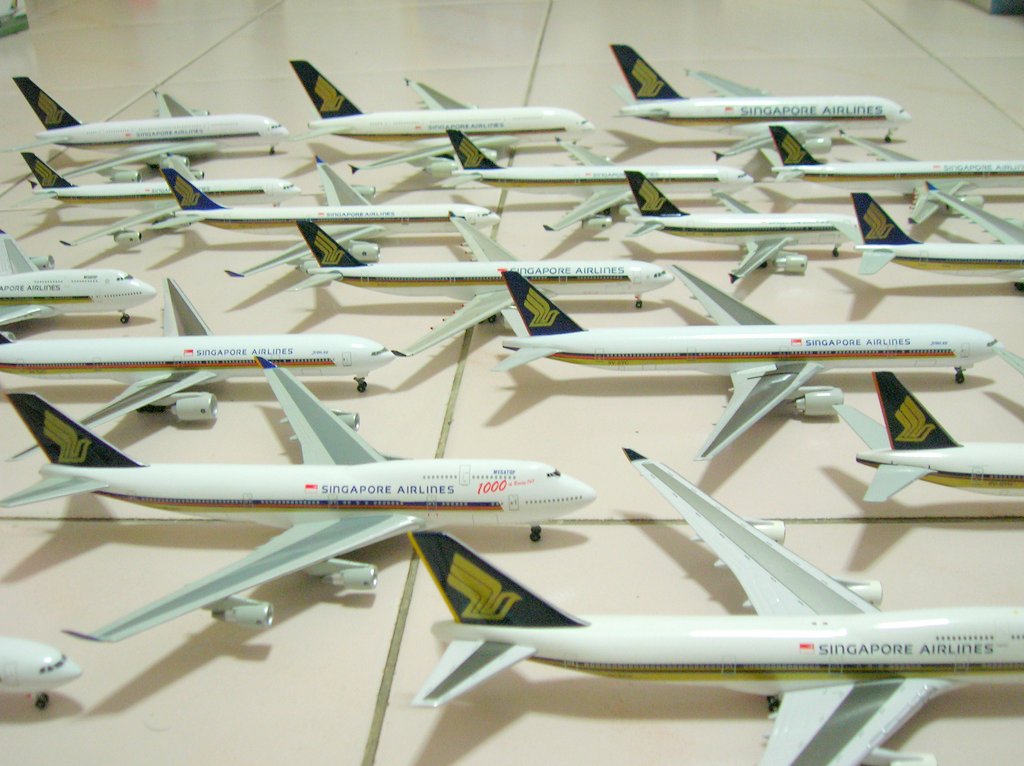The photograph features approximately twenty miniature model airplanes, each bearing the insignia of Singapore Airlines. They are white with blue-tinted tails, all displaying the distinctive blue and yellow Singapore Airlines logo on their sides. The models represent large passenger aircraft from various eras, indicated by slight variations in the logo font and its size on different planes. These models are meticulously arranged on a white tiled floor in about five rows, with each plane positioned very close to the next, yet carefully spaced so that their wings do not overlap. The image focuses solely on the aircraft, with no additional context or objects in the frame.